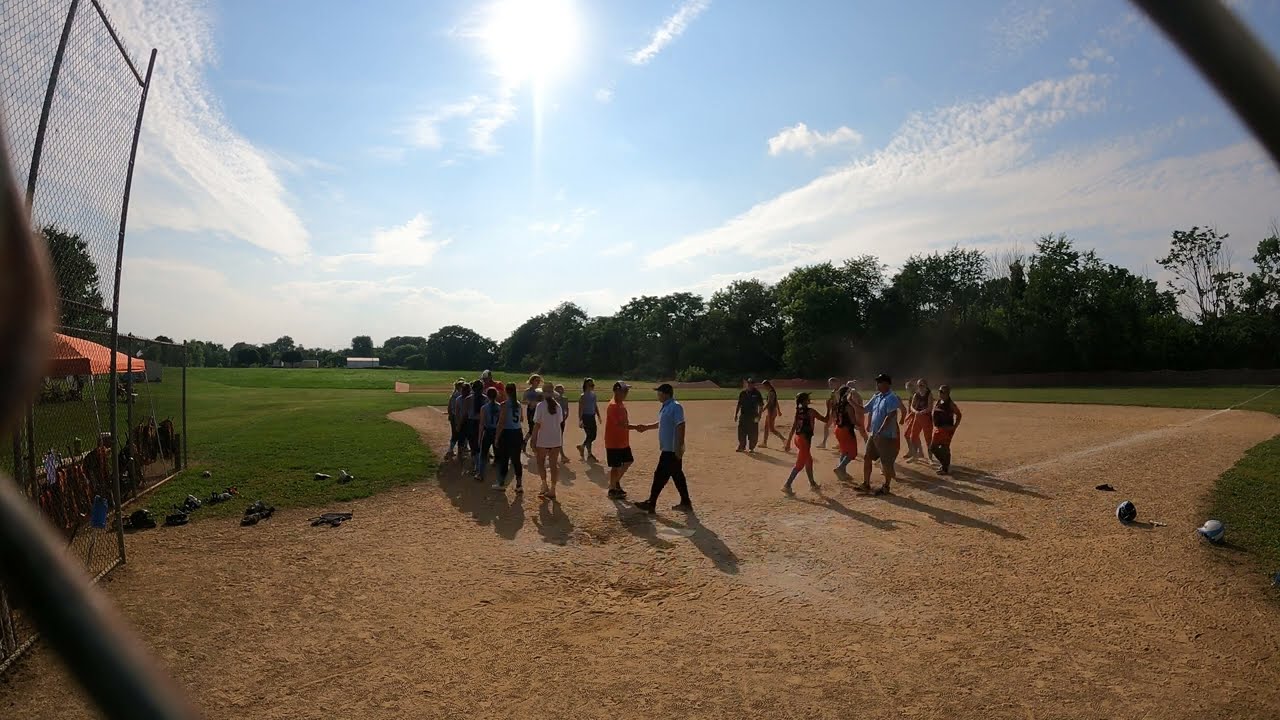The photograph captures a detailed scene of a baseball field at the conclusion of a game, evidenced by players shaking hands in lines near the third and first baselines. The diamond consists of light brown dirt surrounded by a patch of green grass, with the chalk lines faded from play. The sky above is bright and partly cloudy, indicating a warm, sunny day, as some players are wearing shorts and tennis shoes. The teams are distinguishable by different uniforms; one with black shirts and orange pants, the other with bluish-gray shirts and black pants. An umpire in a blue shirt and khaki pants stands at the forefront. To the left of the image, a high chain-link fence and an orange-red umbrella, likely sheltering onlookers, are visible. The background features a tree line and additional green outfield grass, reinforcing the park-like setting. Home plate is faintly visible beneath the dirt, but other bases are not clearly marked. The image appears to have been taken from behind the catcher’s area, as fence wiring dominates the foreground.